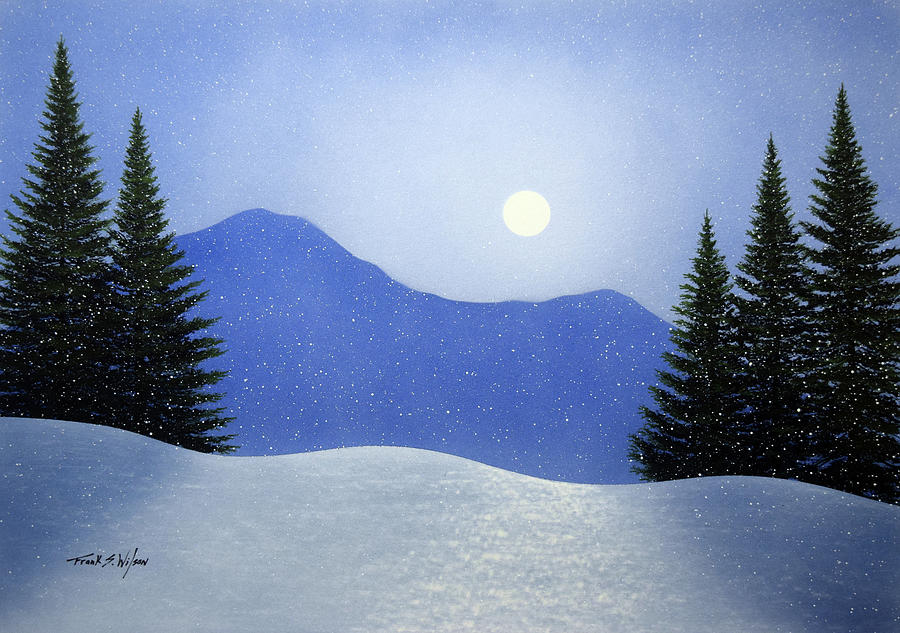This painting by artist Frank S. Wilson, whose signature is located in the bottom left corner, beautifully captures a serene winter night. The scene is set under a softly illuminated blue sky, where a faintly visible sun, partially obscured by fog, casts a muted glow. In the background, dark mountains create a striking contrast to the lighter hues of the sky. The foreground is dominated by a pristine blanket of snow, which is meticulously detailed to emphasize its crispness and depth. Towering pine trees, two on the left and three in the center, frame the composition and draw the eye towards the ethereal sun. Snowflakes gently fall, enhancing the tranquil and festive atmosphere, reminiscent of a quintessential winter wonderland. The painting evokes a strong sense of Christmas and the nostalgic beauty of winter.